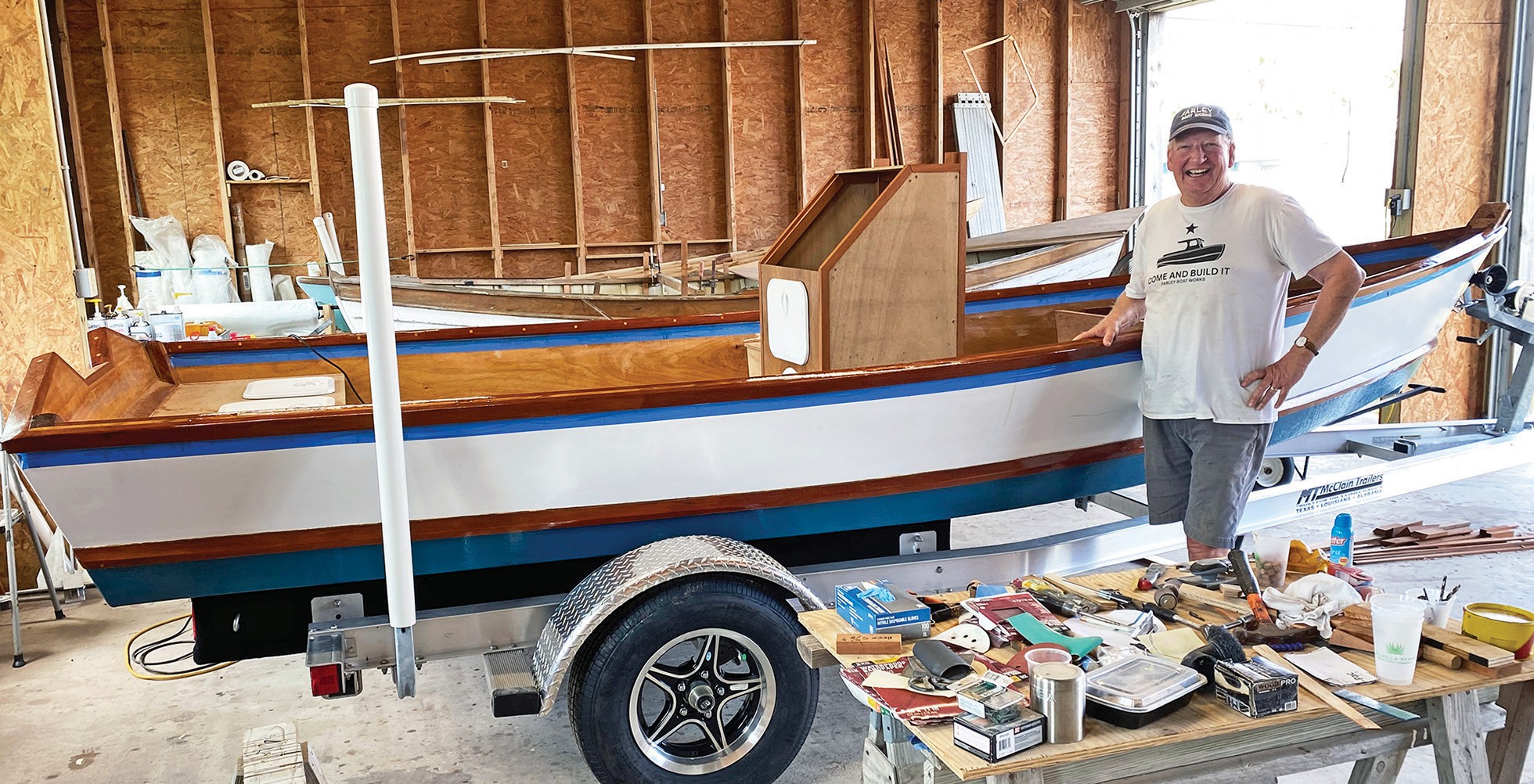The image captures a proud and happy man standing beside a wooden boat that is in the process of being restored. He is wearing a white t-shirt with the inscription "Come and Build It" and a black logo of a boat and star on it. His outfit is completed with a baseball hat that appears to say "sarly" and blue (or gray) shorts, complemented by a watch on his wrist. The man has a big smile on his face, with one hand on his hip and the other resting on the boat. The boat itself is a patriotic combination of red, white, and blue, and it sits on a silver trailer with visible wheels. Surrounding the scene, there is a wooden table covered with various woodworking tools and materials, including screws, a tray, a possible drink container, and a yellow bowl. Also visible is a blue spray. The setting appears to be inside a shop or garage, indicated by the cedar wood walls in the background and the organized workspace. Notably, there is a podium inside the boat, accentuating the meticulous restoration project.